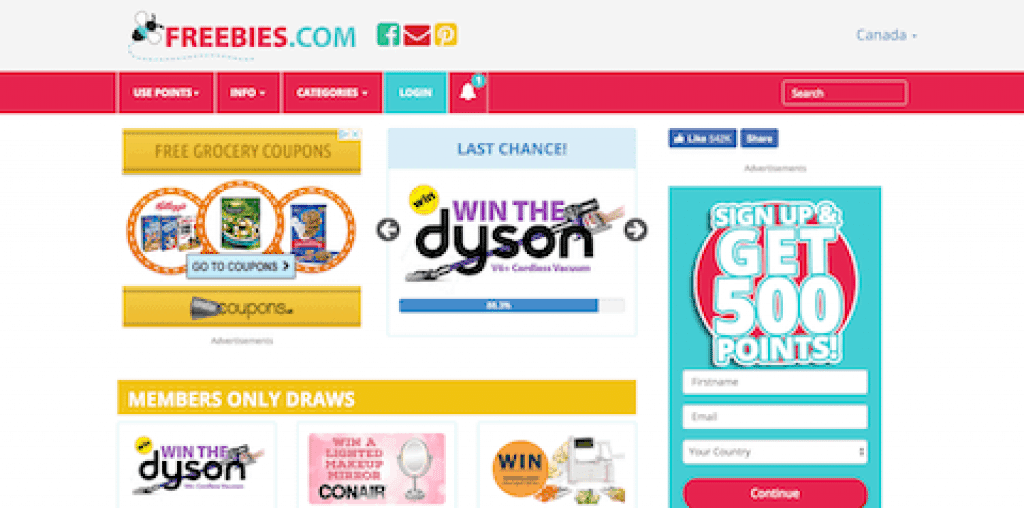The website displayed on the screen is called "freebies.com". At the top of the page, there is a prominent header with the site name "freebies.com". Adjacent to the header are icons for Facebook, email (an envelope icon), and Pinterest, facilitating social media and email interactions. On the far right, a drop-down menu is set to "Canada".

Below the header, a red navigation bar with white text spans the width of the page, featuring several drop-down menus: "Use Points", "Info", and "Categories", each marked with a down arrow to indicate additional options. Also within the navigation bar is a "Login" button with a teal background, and to its right, an alert button displaying a notification with the number 1 in teal. Further right, there is a search button for user queries.

The central portion of the page showcases multiple sweepstakes entries. One highlights the chance to get free grocery coupons, while another offers a chance to win a Dyson product. A header titled "Members Only Draws" introduces three specific sweepstakes: one for winning a Dyson, a second for winning a Conair lighted makeup mirror, and a third partially obscured entry simply labeled "Win".

On the far right side of the page, there is a large, attention-grabbing graphic encouraging visitors to "Sign up and get 500 points." Below this graphic, users are prompted to enter their first name, email, and country, followed by a "Continue" button to advance the sign-up process.